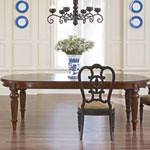This photograph depicts a cozy, elegantly decorated dining room. The room has a white paneled wall with light vertical lines and features a prominent window in the center that's letting through a soft light, softly illuminating the space through see-through curtains. On either side of the window, there are two decorative plates arranged in pairs — one pair on the top left and the other on the top right. These plates have blue edges and white centers, adding a touch of color to the otherwise neutral walls.

The centerpiece of the room is a round wooden dining table with a glossy finish that reflects light beautifully. On this table stands a striking blue and white vase filled with green foliage and white flowers, creating an inviting focal point. Directly in front of the table, facing the camera, is a wooden chair with an ornate backrest and a tan padded seat. Another chair is partially visible off to the side.

Overhead, a chandelier with ornate arms and light fixtures adds a touch of sophistication to the room. The floor is a well-polished hardwood, adding warmth to the space and reflecting light from the window, accentuating the room's clean and bright atmosphere. The overall setup exudes a timeless charm and a well-appointed aesthetic perfect for elegant gatherings.